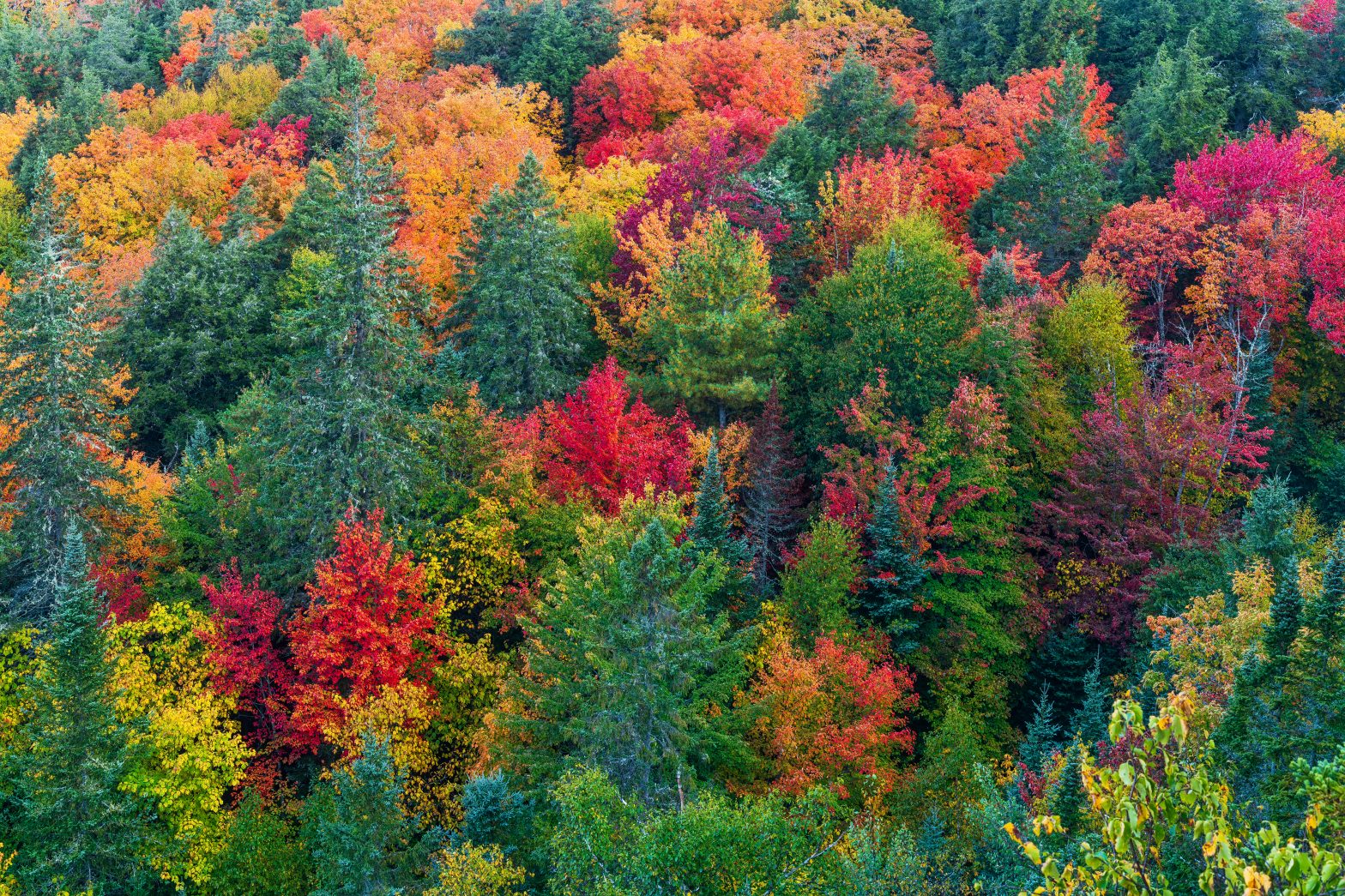The image is a stunning aerial view of a dense, vibrant forest awash with the colors of late autumn. Taken from high above, the overlook captures a rich tapestry of trees - a harmonious blend of towering pines and robust hardwoods like oaks and maples. The coniferous evergreens maintain their steadfast green, providing a lush backdrop to the explosion of fall colors. The deciduous trees are in the midst of their seasonal transformation, showcasing an array of deeply saturated hues: dark burgundy reds, bright oranges, yellows, and even some magentas. The colors create a mesmerizing gradient, from vivid pinkish-reds to burnt oranges, illustrating the forest's breathtaking abundance. Despite some trees appearing thin and with leaves that are starting to yellow, the overall scene is one of magnificent, almost surreal, beauty, reminiscent of an idyllic autumn setting often depicted in classic films. The dense concentration of foliage makes it difficult to distinguish individual trees, emphasizing the forest's vastness and the sheer volume of life it supports.